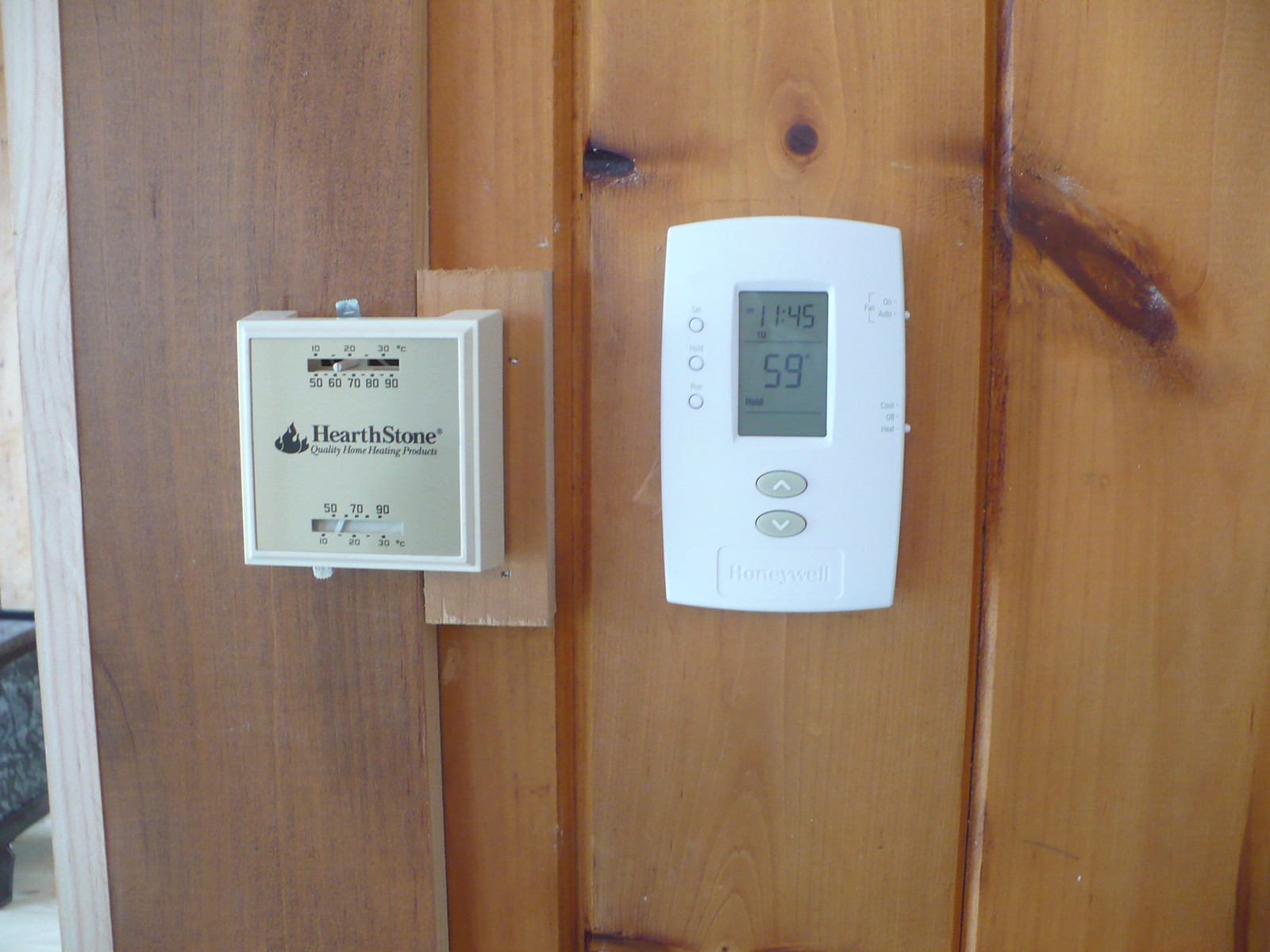A landscape-oriented photograph captures the interior wall of a home, showcasing a light wood-paneled surface with distinct grain patterns on each plank. Centrally mounted on the wall are two temperature gauges. The left gauge is square-shaped, labeled "Hearthstone" in black letters with a logo, and displays a reading close to 78 degrees, indicated by a silver marker. To the right, the thermometer is rectangular and white, featuring an LCD screen that shows a time of 11:45 and a temperature reading of 59 degrees. Below the screen are two gray buttons, one with an upward-pointing arrow and the other with a downward-pointing arrow.